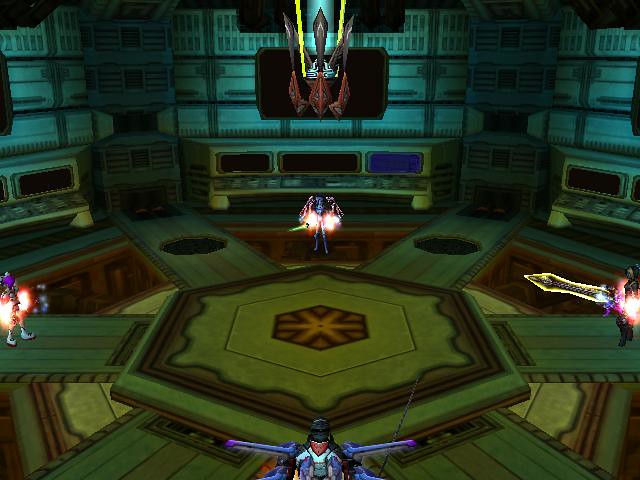The image depicts a still from a video game, featuring a dark, moody environment dominated by deep green and turquoise hues. The screen is divided into four quadrants, each showcasing a different player character, all facing towards the center. There's a hanging light fixture casting a dim glow from the ceiling, adding to the ominous atmosphere. The character in the right quadrant wields a sword, while the character positioned at the bottom center appears to have wings. Notably, the image contains no text or other on-screen indicators.